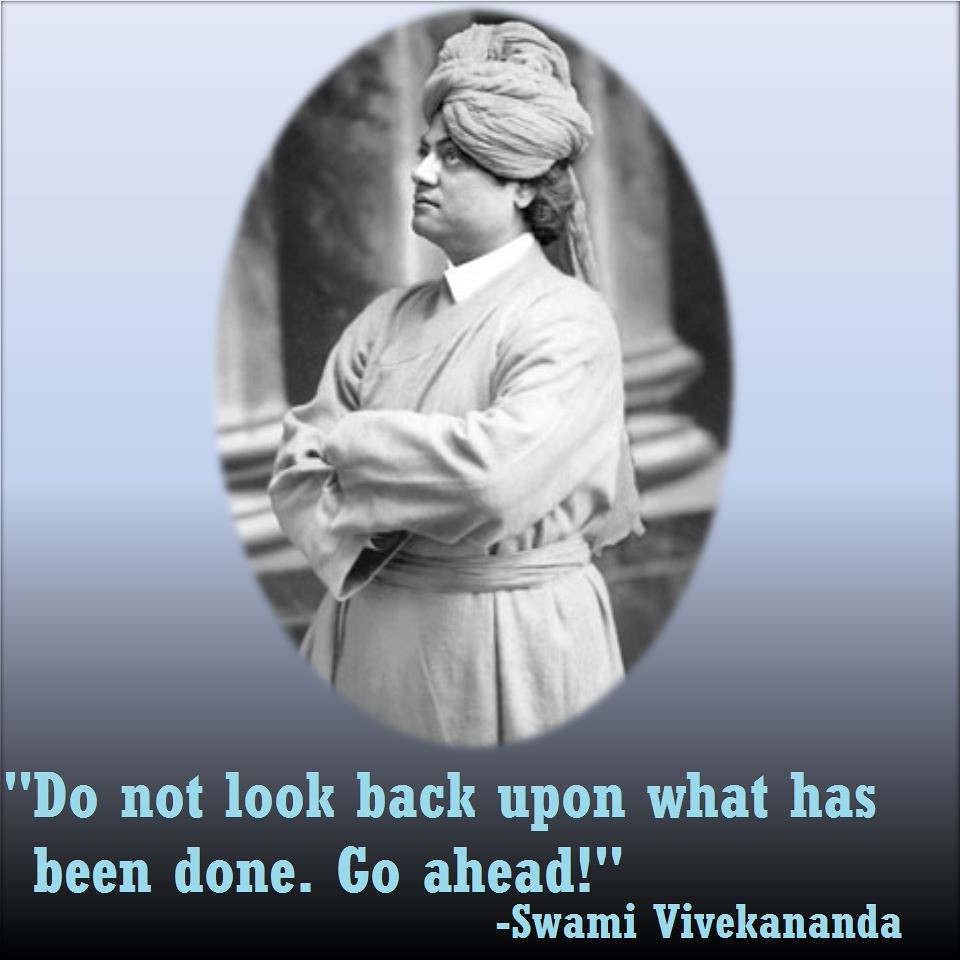The image features a black-and-white, oval-shaped portrait of Swami Vivekananda, captured in front of what appear to be marble columns. He stands with his arms crossed, looking slightly upward, his left side turned towards the camera. Swami Vivekananda is dressed in a turban and a long robe with wide sleeves, his hands tucked into the sleeves across his chest. The background surrounding the oval portrait has a gradient transitioning from black at the bottom to white at the top with a subtle bluish tint. Beneath the image is a quote in blue text that reads, "Do not look back upon what has been done. Go ahead!" followed by his name, Swami Vivekananda.